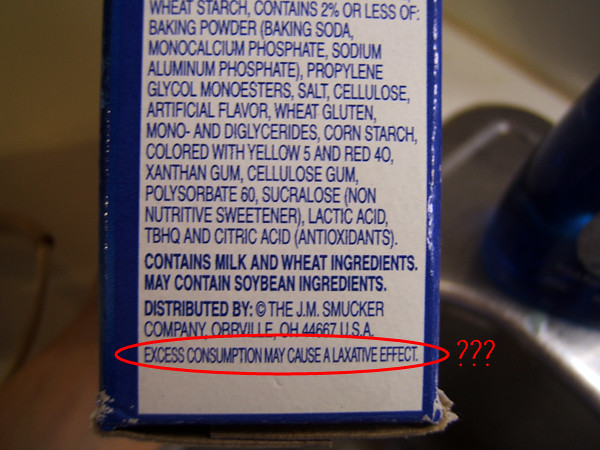A photograph captures a hand holding a box of macaroni over a sink. The box features a detailed ingredients list, including wheat starch, baking powder (comprising baking soda, monocalcium phosphate, and sodium aluminum phosphate), propylene glycol monoesters, salt, cellulose, artificial flavor, wheat gluten, and mono and diglycerides. An arm is visible at the bottom left corner of the image, suggesting someone is preparing to use the contents.